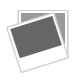The image is a photo of a magazine front cover with a cartoon drawing of a male figure who has slipped on a banana peel and is now tumbling headfirst onto a concrete sidewalk. The magazine title "Bananas" is boldly written in yellow bubble text. Below it, a playful tagline reads, "We Trip Up the Fall Guy!" The character is drawn with a button nose, brown hair, and is outfitted in a distinctive leather brown jacket adorned with stars on the back, blue jeans, and cowboy boots. The background of the cover features a soft gray and vibrant orange, and though there is unreadable text in the upper right-hand corner, the primary focus is on the humorously depicted scene. The setting suggests an outdoor, daytime environment capturing the moment of the mishap. The attention to detail, from the fallen banana peel to the character's expressive pose with legs up in the air and hands bracing for impact, adds a comic, lively feel to the magazine cover.